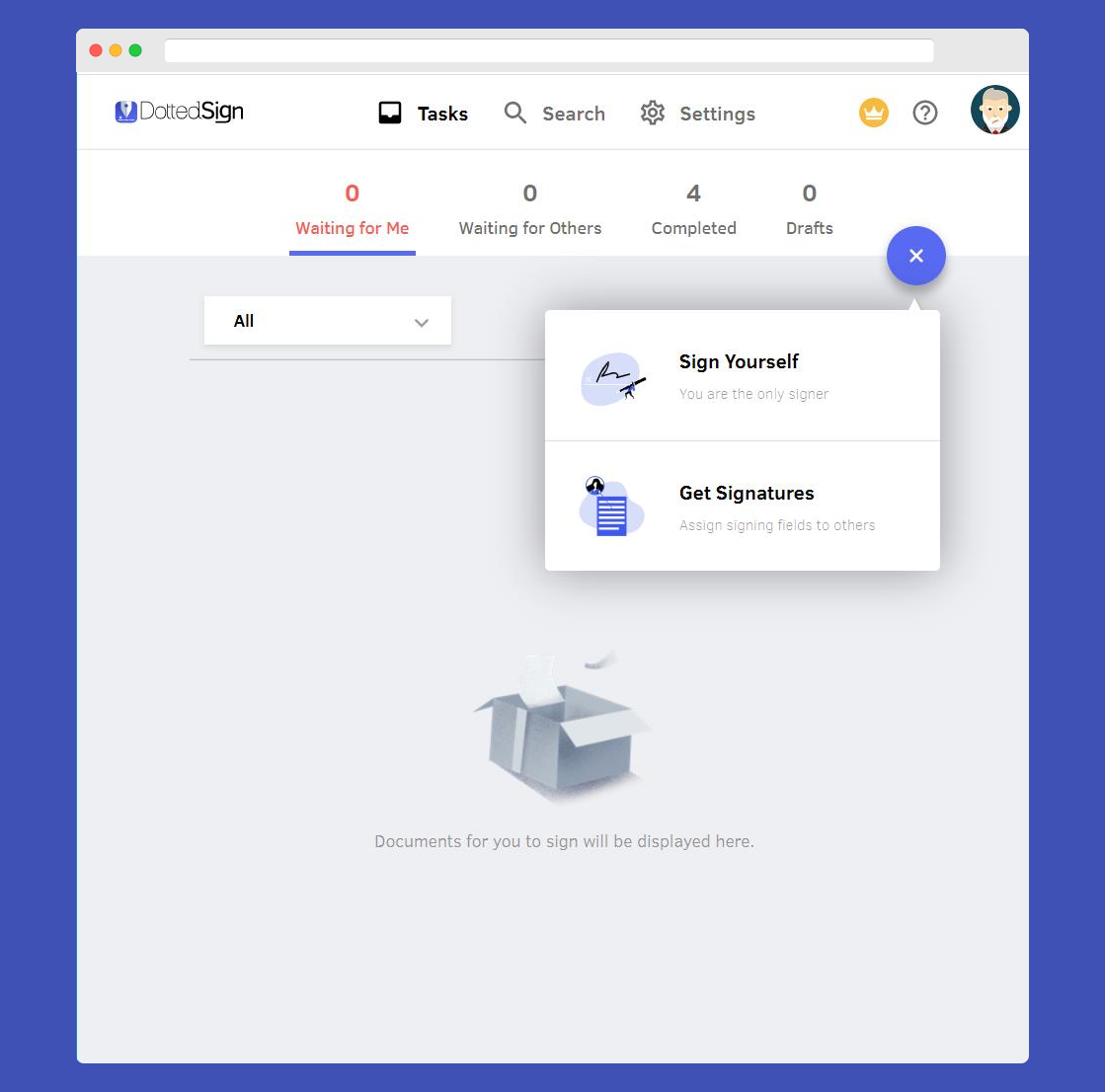A computer window with a minimalistic user interface is displayed. At the top-left corner, there are three colored dots: red, yellow, and green, representing the standard window control buttons (close, minimize, and maximize). Adjacent to these is an empty search bar. 

Beneath the search bar is a blue logo followed by the text "dotted sign," where "dotted" is in gray and "sign" is in bold black letters. Below this is a navigation menu featuring the bold black word "Tasks." Accompanying this section are icons: a magnifying glass for search, a gear for settings, a gold crown button, a question mark, and an avatar of an elderly man with glasses situated on the far right.

Under this menu, the interface shows several status indicators: "Waiting for me" in red lettering, "Waiting for others," "Completed," and "0 drafts." 

A tab labeled "All" is visible with a bar beside it and a drop-down menu, currently not expanded. Beside this are options for signing: "Sign yourself" (indicating you are the only signer) or "Get signature" (assigning signing fields to others). A blue "X" in a blue circle icon accompanies these options.

At the bottom, there is an open box icon with papers spilling out, accompanied by the text "Documents for you to sign will be displayed here."